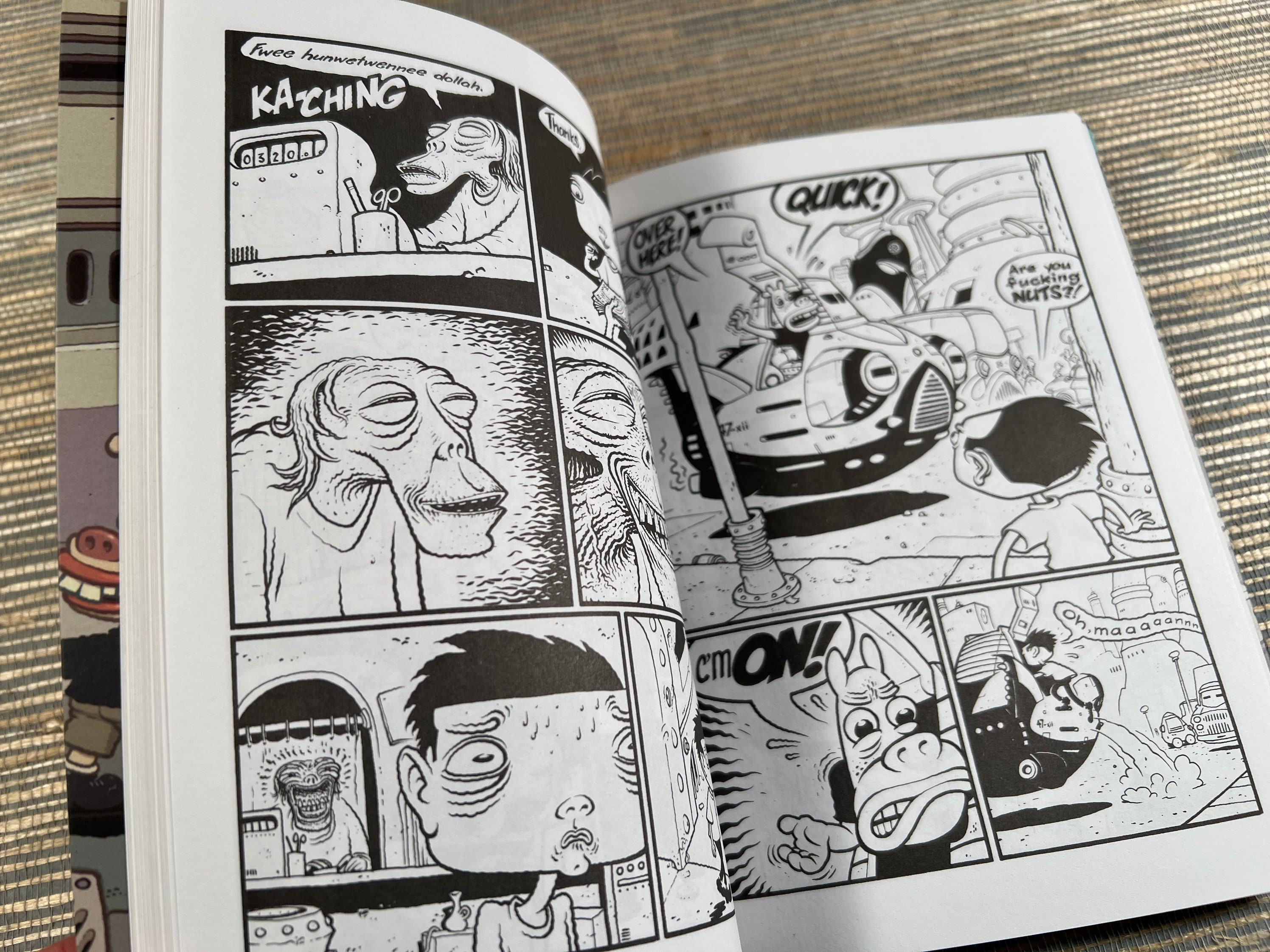This photograph captures a partially open black-and-white comic book, showcasing its unique, 90s Nickelodeon-like art style with graphics reminiscent of Rugrats or As Told By Ginger. The comic features various panels: one depicts a long-faced, alien-looking creature with round, protruding eyes, while another shows a fearful humanoid boy. On the left side, an old man with a gaunt face, seemingly running a cash register, is shown yelling with exaggerated expressions, making fun of a kid and mentioning a figure like "$300" or "$500" in a heavy accent. On the right side, a comical spacecraft appears to be flying through the street, accompanied by dialogue bubbles with expletives, where the child exclaims, "Are you effing nuts?" Another panel hints at a pig-like or hippo-like creature urging the boy to hop into the vehicle, adding a touch of surreal humor typical of comic book narratives.